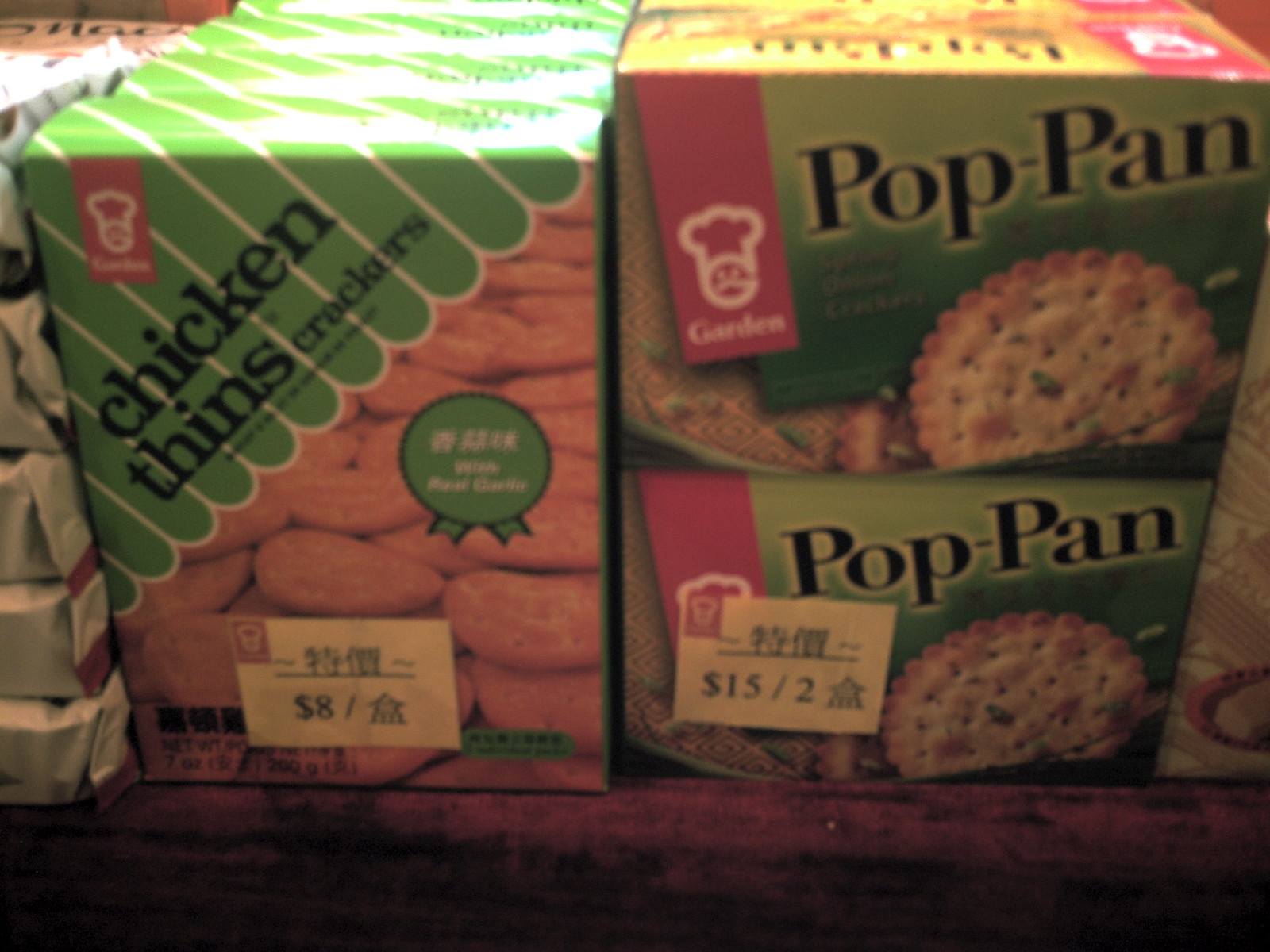The photograph is a slightly blurry and unfocused color snapshot, capturing a grocery store shelf stocked with various food items. Centered in the image are two clear items: a box of Chicken Thins crackers and a package of Pop Pan crackers. The Chicken Thins box, positioned just left of center, stands vertically and features a light yellow label adorned with Asian script and a price tag of $8. To its immediate right is the Pop Pan box, placed horizontally and also featuring Asian text with a price label indicating $15 for two. The green boxes of Pop Pan crackers display images of the crackers themselves. Behind these primary items, the shelf is filled with a miscellany of stacked boxes, while the far left side of the image shows a smaller, more organized stack of goods. The entire scene is bathed in a tungsten tint, lending a warm cast to the photograph. Various other pictures and small text can be seen on the boxes, adding to the visual clutter.